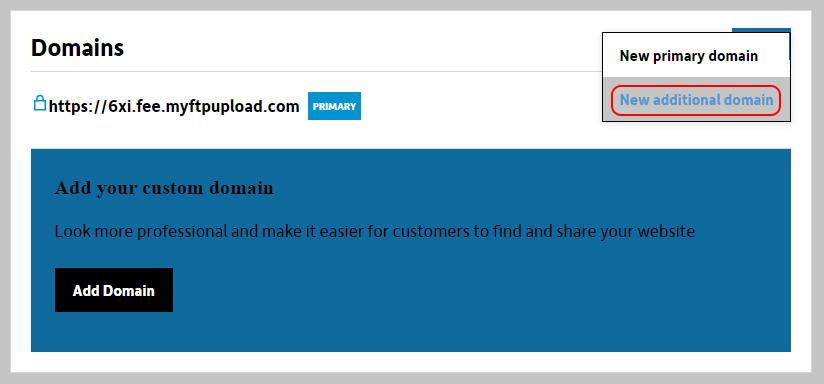This screenshot, likely taken from a laptop, displays a pop-up window. It features a white rectangular interface outlined by a gray border. At the top left of this rectangle, "Domains" is prominently written in thick black font. Adjacent to it is a light blue lock icon, accompanied by the URL "https://6zi.fi.myftpupload.com." 

Below this, there is a blue rectangle containing the word "Primary" in white font. To the far right, black text reads "New Primary Domain," followed by "New Additional Domain" in blue font. This latter phrase is enclosed in a red rectangle.

Further down, a large blue rectangle is present with the bold, black text "Add Your Custom Domain." Beneath this, in slightly less bold font, the message "Look professional and make it easier for customers to find and share your website" is displayed. Finally, a black rectangle at the bottom bears the white text "Add Domain."